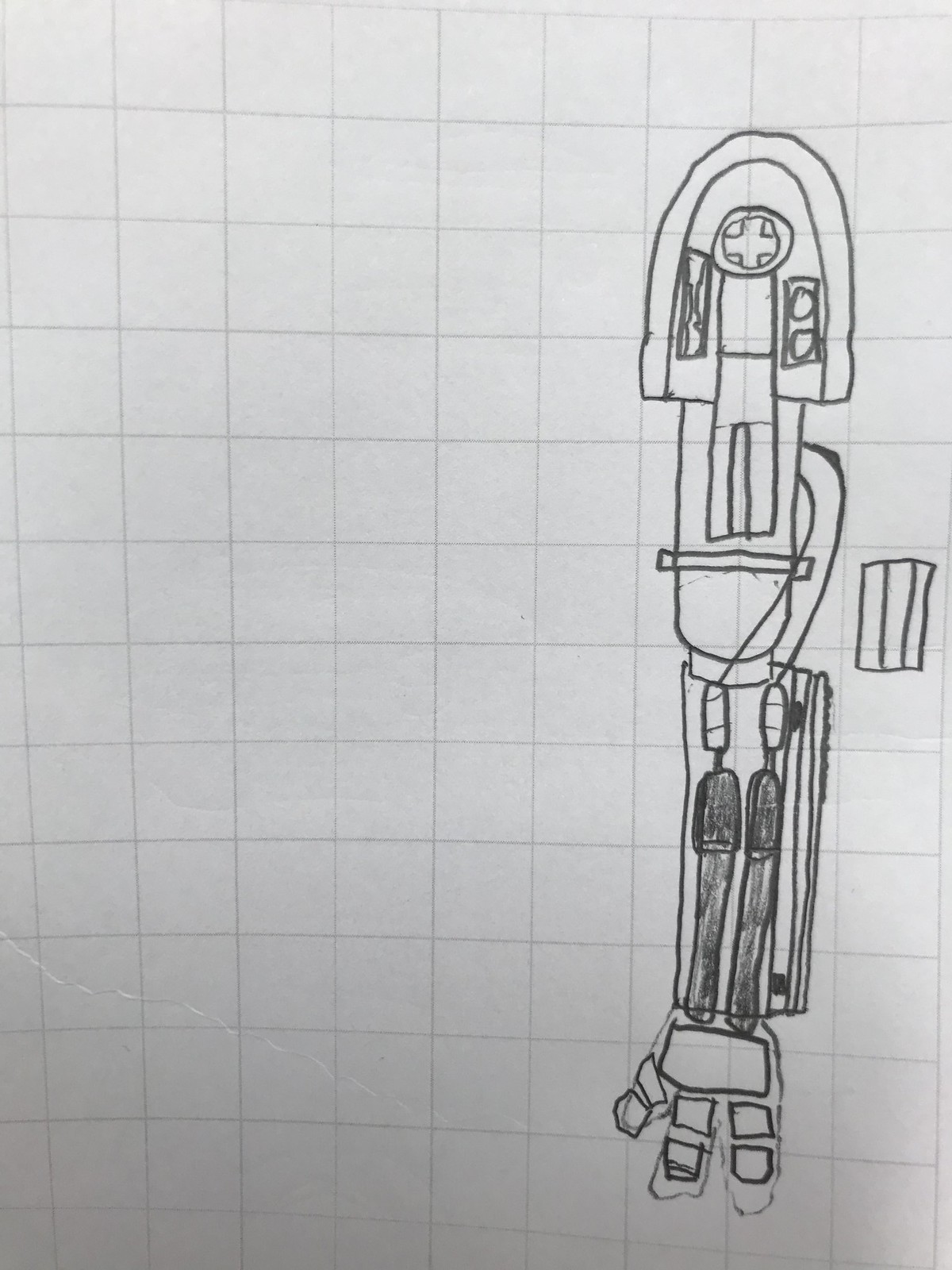This is a photograph of a detailed pencil drawing on graph paper, featuring a complex amalgamation of a mechanical arm and a creature that appears part vacuum cleaner, part human. The graph paper has gray lines on a white background, with each square measuring roughly half an inch to an inch. The drawing occupies the right side of the paper and consists of various elements, highlighting the creator's intricate sense of detail.

The mechanical arm, vertically long and occupying 11 squares, showcases three fingers, each with two joints, and is drawn with additional mechanical components such as wires near the elbow, suggesting a hydraulic system. At the top of the arm, near the shoulder joint, is a cross inside a circle, reminiscent of a patch or badge. 

Intriguingly, the torso of this creature integrates humanoid elements, suggesting a smaller individual trapped inside. Extending from this torso is a hose-like structure leading to the lower part of the creature. This lower segment resembles a bag enveloping two legs that merge into a single foot with three toes. In the background, there is a box divided into three segments, adding to the overall complexity and intrigue of the drawing. The entire piece, while not over-detailed, exudes a creative precision often seen in middle school or high school-level artwork.